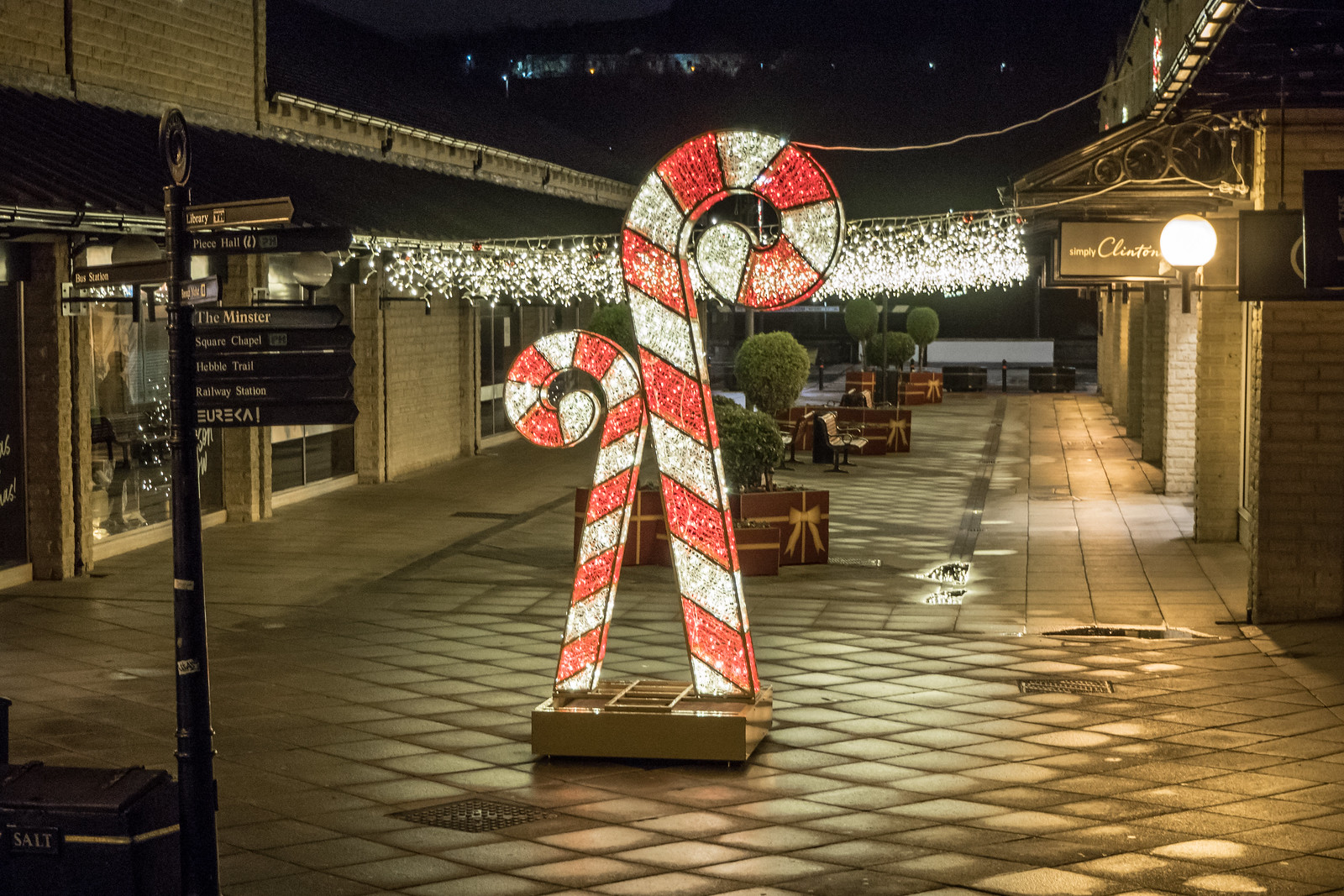In this atmospheric holiday night scene, we see a well-lit outdoor shopping mall adorned with festive decorations. At the forefront, two candy cane decorations stand on a brown pedestal—the larger on the right, the smaller on the left—each brilliantly illuminated in red and white with a blue outline that gives them a sparkling appearance. The walkway, made of beige, checkered stone blocks, stretches into the distance, flanked by storefronts on both sides.

Near the candy canes, three distinct plant arrangements housed in elegant, black-and-gold plant holders are visible, each adorned with decorative ribbons. Behind the candy canes, a string of twinkling white Christmas lights hangs between buildings, adding to the festive ambiance. Green shrubbery in wooden crates with bows adds a touch of nature amidst the urban setting.

On the left side of the image, a directional sign in the closest foreground lists locations such as Minster Square Chapel, Hebel Trail Railway Station, and Eureka. Floor-level lighting casts a warm glow, highlighting the pathway and the entrances to various shops. The sky overhead is an inky, almost pitch-black, which starkly contrasts with the colorful, illuminated scene below.